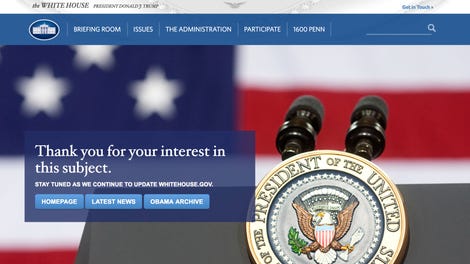The screenshot captures the homepage of the White House website. At the top, a navigation bar prominently displays "The White House" along with a blue background featuring an outline of the White House itself. Adjacent to this logo are several navigation tabs labeled "Briefing Room," "Issues," "The Administration," "Participants," and "1600 Penn." Additionally, there's a search bar to the right for site-wide searches.

Beneath the top bar, the background image partially showcases the American flag, revealing three stars in the upper left corner and portions of the red and white stripes. Superimposed on this background is a blue block containing text in white that reads, "Thank you for your interest in this subject." Below this, a message states, "Stay tuned as we continue to update whitehouse.gov." 

Further down, there are clickable options in light blue font for "Home Page," "Latest News," and "Obama Archive." Adjacent to these links, an image shows the top of a podium equipped with two microphones. At the bottom of the screenshot, the Seal of the President of the United States is prominently displayed.